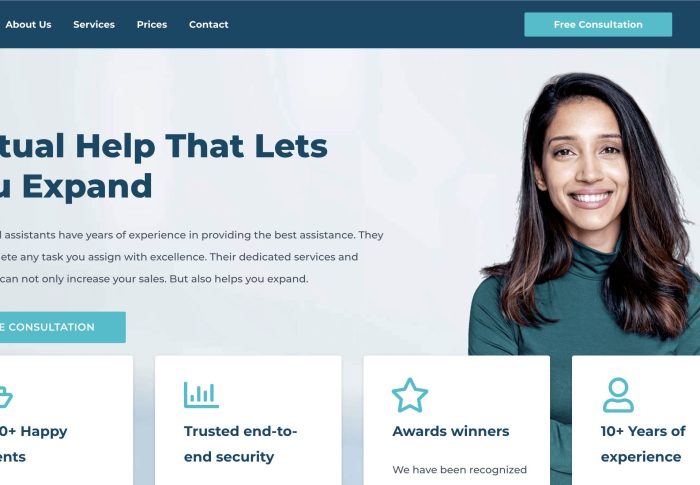The website features a clean and structured layout with a light gray background. At the top, there are four main categories in white text arranged from left to right: "About Us," "Services," "Prices," and "Contact." In the top right corner, there is a light blue rectangle with the text "Free Consultation" centered within it.

Directly below the main navigation bar, there is partially obscured text that includes the words "T-U-A-L," "help," "let's," and "expand." Further down, a section highlights the company's expertise: "Assistants have years of experience in providing the best assistance." The fully visible text captures the key points: "They handle any task you assign with excellence. Their dedicated services can not only increase your sales but also help you expand."

To the right of this content, an image features a woman with black hair wearing a dark green shirt. She is smiling directly at the camera, giving a friendly and approachable impression from the front view perspective.

Toward the bottom of the page, there is another light blue rectangle with the word "Consultation." The website concludes with four distinct white squares, each containing succinct messages: "Happy Clients," "Trusted End-to-End Security," "Award Winners," and "10 Years of Experience," showcasing the company's achievements and client satisfaction.